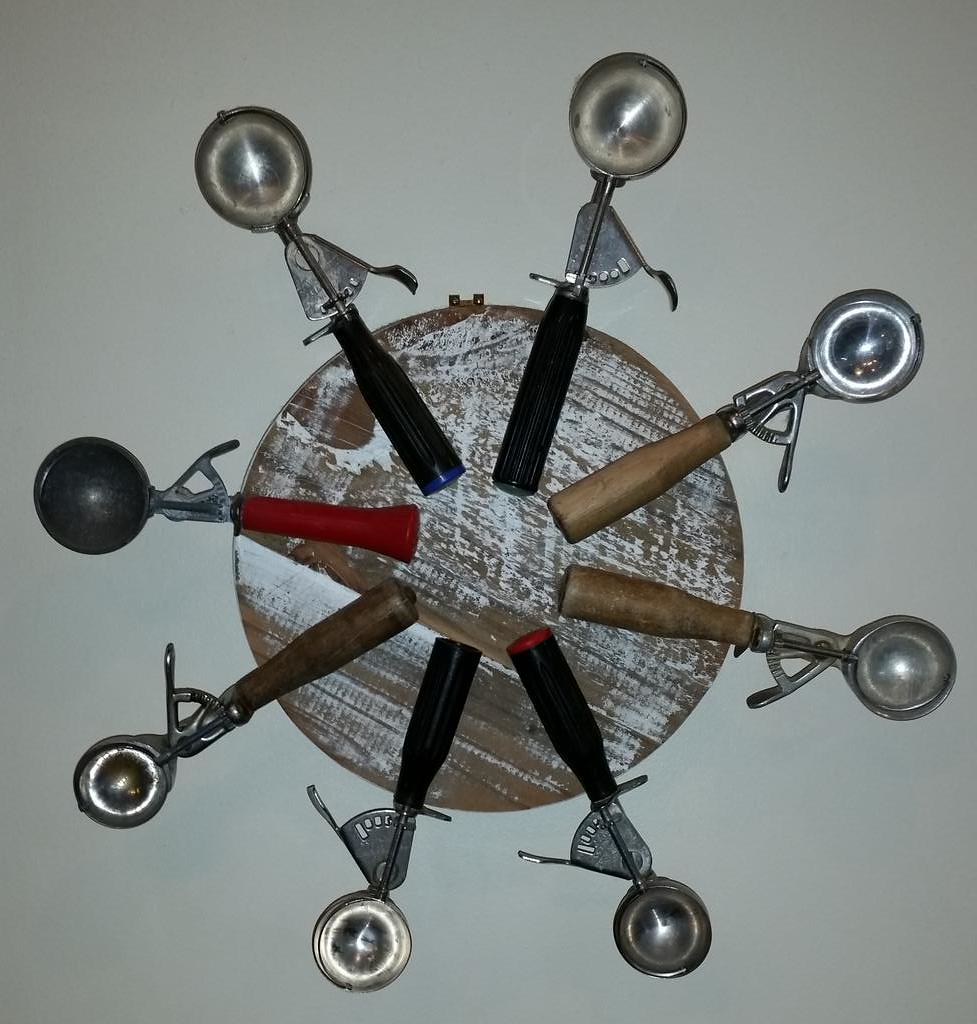This color photograph, taken with flash, features eight vintage ice cream scoops arranged in a circular pattern, resembling spokes in a star. The scoops converge at the center, where the handles meet to form a circle. Each scoop has an old, scratched, and faded metallic appearance, equipped with thumb-operated squeezing mechanisms. The handles vary in material, with some fashioned from plastic and others from wood; their colors include black, brown, dark brown, and red. Notably, the scoop with the red handle has a unique black metal scoop instead of the standard silver. These ice cream scoops are displayed on a brown wooden disc that appears to have been lightly brushed with white paint, giving it a worn and rustic look. This entire setup rests on a white surface. There is no writing, and the background is uniformly gray, providing a simple, unobtrusive backdrop for the antique tools.